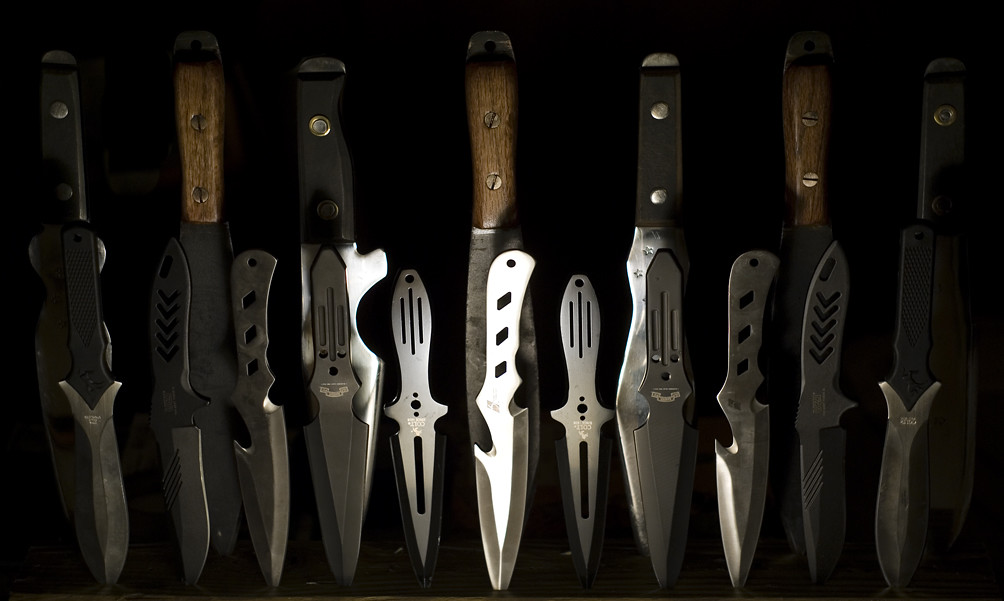This color photograph, set against a completely black background, showcases an intriguing collection of ornamental knives. There are approximately 10 to 12 knives, vividly illuminated to emphasize their craftsmanship. The knives are arranged vertically, with their sharp points embedded in what appears to be a table. 

The arrangement follows a consistent pattern of alternating black and brown handles, with each handle crowned with a silver top, possibly resembling nuts. Among the handles, some are made of wood, others of metal, and they feature intricate silver carvings. Notably, there also appears to be a blade without a handle situated in the middle of the arrangement.

Each knife boasts a thick silver blade, some adorned with ridges or vertical lines, showcasing meticulous detailing. The knives vary in size, from long elegant blades to smaller, more compact ones, and they seem to include different types, possibly for throwing or as culinary tools, though none have serrated edges. The contrast between the illuminated blades and the dark background highlights the striking design and sharpness of these knives, creating a visually compelling image.